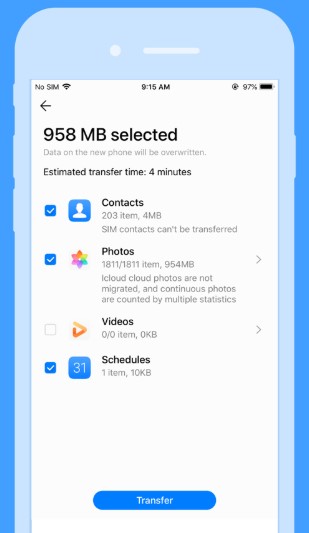The image depicts a screenshot of a cell phone interface that appears somewhat simulated given its light blue outline, with a darker blue border encasing it. The screen displays a data transfer process.

The top section of the screen indicates various statuses: "No SIM," Wi-Fi icon, "9:15 a.m.," and "97% battery." Below this, a back arrow is visible alongside the text "958 MB selected." A warning notes, "Data on the new phone will be overwritten," with an estimated transfer time of 4 minutes.

In the data breakdown:
- **Contacts**: 203 items totaling 4 MB (with a note that SIM contacts cannot be transferred).
- **Photos**: 1811 items totaling 954 MB (yet indicating that iCloud photos are not migrated and continuous photos are handled by different statistics).
- **Video**: 0 items totaling 0 KB.
- **Schedule**: 1 item totaling 10 KB.

Each category - Contacts, Photos, and Schedule - is marked with a filled blue checkbox featuring a white checkmark, indicating they have been selected for transfer. At the bottom of the screen is a prominent blue button labeled "Transfer" in white text.

The color palette used in this interface includes shades of blue, orange, yellow, green, purple, red, white, black, and gray.